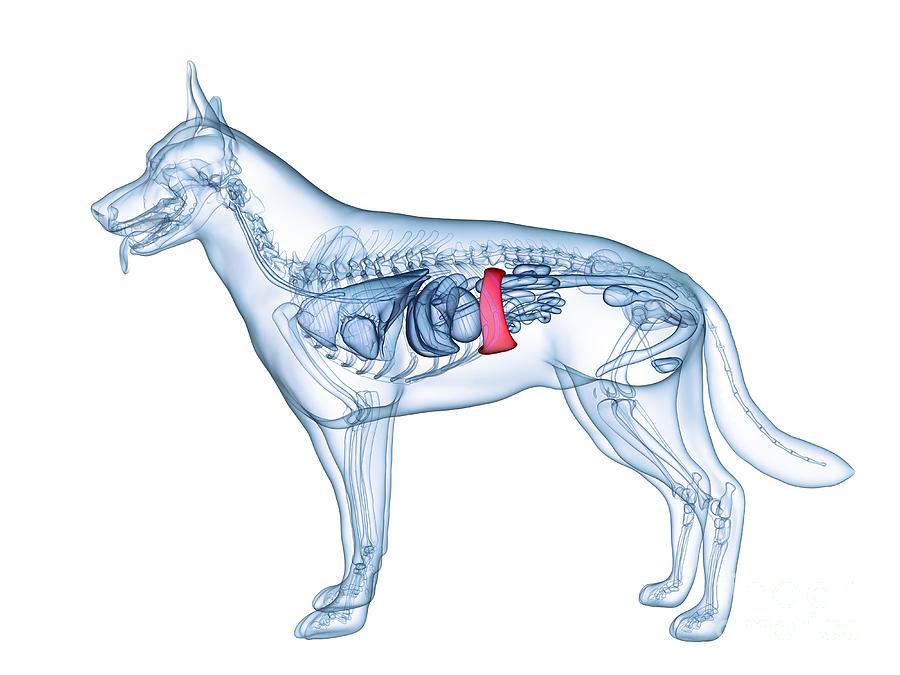In this digital image of a dog set against a white background, the animal appears almost transparent, created in blue and gray hues to resemble an x-ray. The side-view composition shows the dog standing tall and facing left with its tongue hanging out, ears perked, and nose visible. Through the semi-transparent outer body, a detailed internal anatomy is revealed, including the skull, spine, chest bone, and bones running down the legs to the paws and tail. Within this skeletal framework, the dog's internal organs are depicted, such as the heart, lungs, stomach, spleen, kidneys, and intestines, with most rendered in black and white tones except for one organ highlighted in red. The overall effect provides a comprehensive view of the dog's exterior and interior anatomy, blending artistic digital imaging with the aesthetic of medical x-ray imagery.